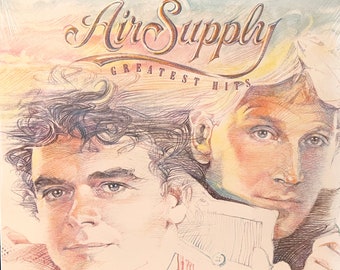This album cover of Air Supply’s “Greatest Hits” prominently features a colored pencil sketch of the two main singers. Both men's faces are shown in a close-up, headshot style against a backdrop of very light, almost pastel colors, which include shades of tan, yellow, peach, light pink, light blue, and beige that blend subtly with the men’s complexions. The man in the foreground has darker, wavy hair and brown eyes, while the slightly backgrounded figure has shorter, straight blonde hair and blue eyes. The title "Air Supply Greatest Hits" is written in brown text that complements the light background hues. The overall aesthetic is reminiscent of a 90s movie cover and gives a nostalgic vibe without appearing strictly contemporary or old-fashioned.